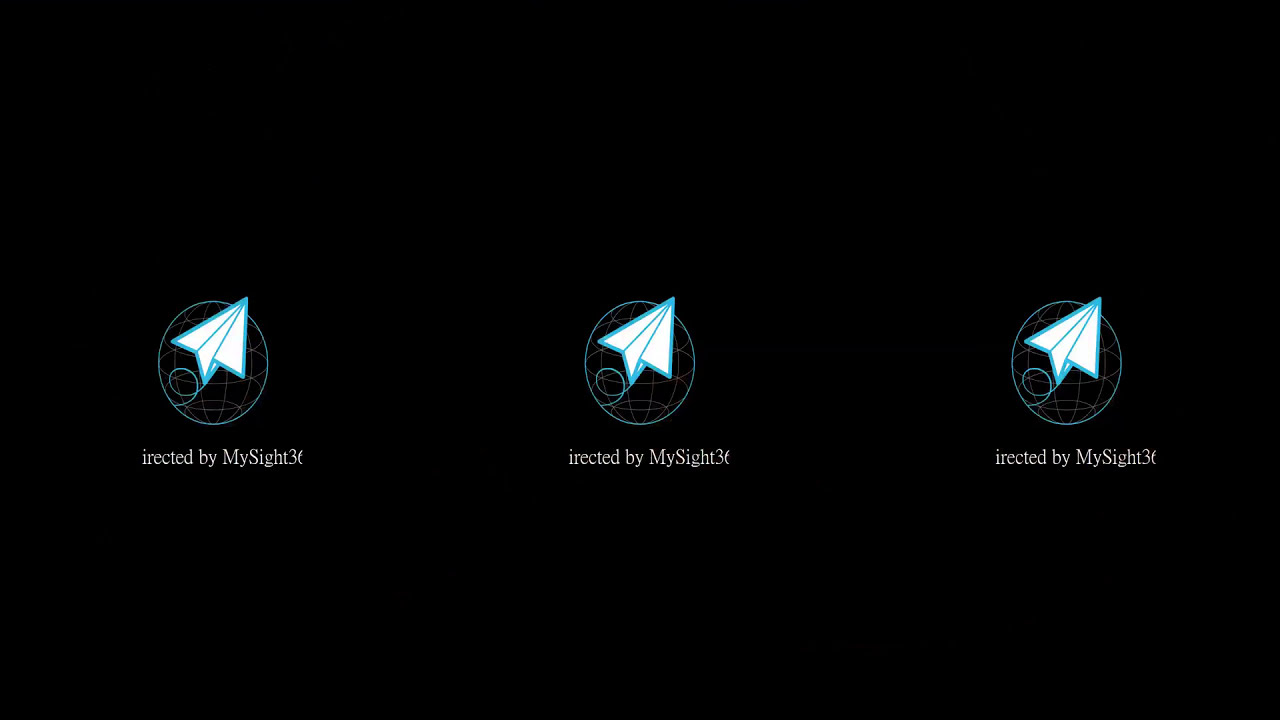The image is a rectangular composition with a solid black background. In the center are three identical emblems, evenly spaced from left to right. Each emblem features a paper airplane illustration with detailed blue lines highlighting the folds. A blue, twirling line extends from the back of the plane, looping to the left, rising up, then down to the right, and connecting to a near-complete circle around the airplane—leaving only the tip of the plane protruding upwards slightly to the right.

Each emblem is further detailed with a teal circle containing a light brown or light gray grid pattern, reminiscent of a globe. The paper airplane is white with a light blue border. Below each emblem, in white font, the text partially reads "erected by MySite36," although some parts are cut off. The overall image gives a minimalist and uniform visual experience, with all other elements surrounding the emblems rendered in plain black.